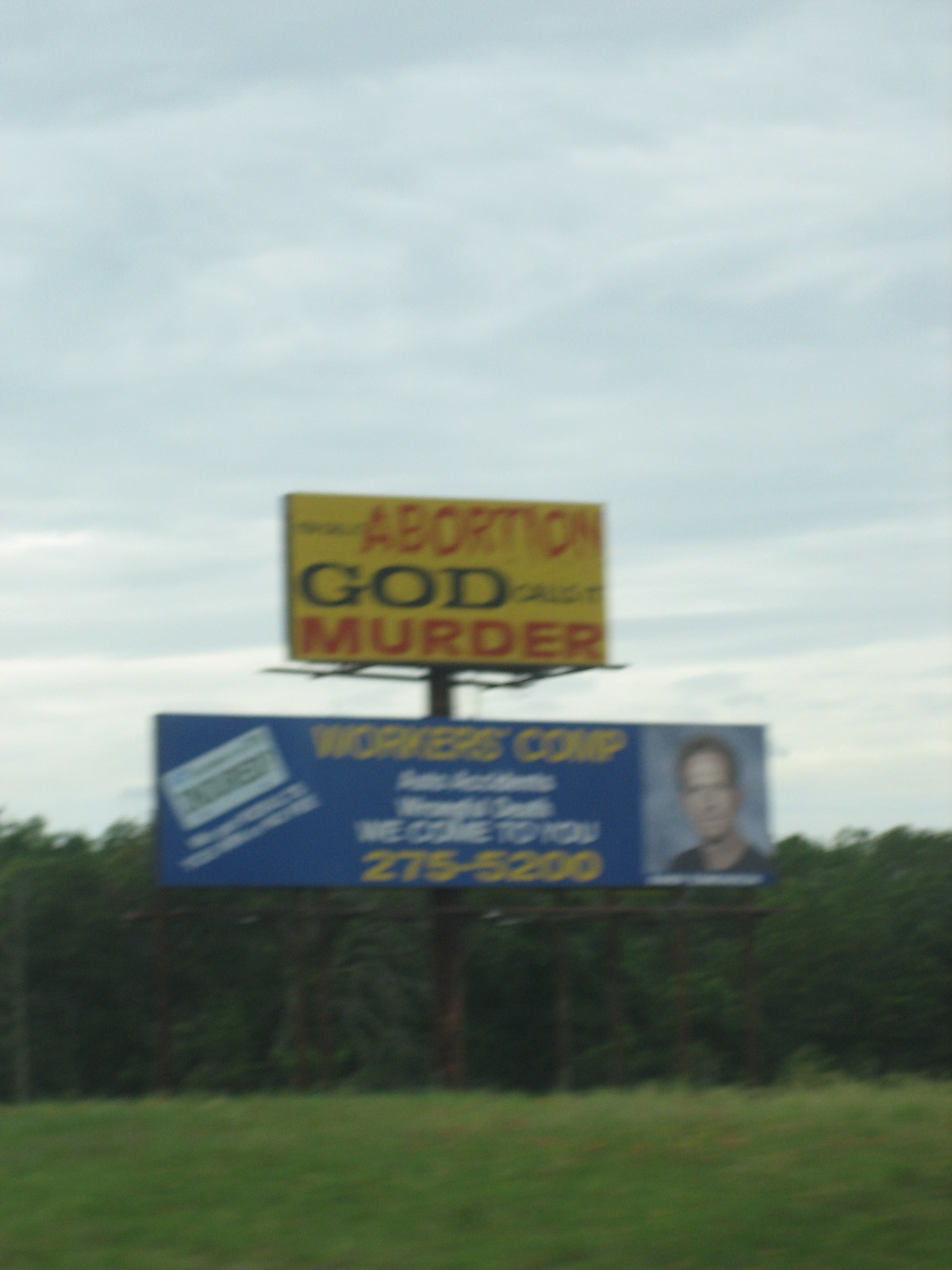The image captures a scene with two billboards mounted on a single pole, visible just above a dense tree line that covers the lower quarter of the image. At the bottom of the image, there's a dark green grass lawn in the foreground. The larger, lower billboard is predominantly blue on the left side and notably blurry, making its text largely illegible. However, partial details can be inferred: it features a yellow and white text with phrases like "Workman's Comp" and "we come to you," along with a telephone number ending in "5 2 0 0." The right side of this billboard displays a blurry image of a man, possibly a white male with thinning hair, seemingly wearing a black t-shirt, which contrasts with the expectation of a more formal attire for such advertisements.

Above this is a smaller but clearer yellow billboard with a stark, controversial message. It carries large, easily readable red letters at the top spelling "Abortion," followed by "God" in bold black letters in the middle, and "Murder" in red letters at the bottom. Additional smaller text before "God" reads, "calls it," suggesting the full message is "You call it Abortion, God calls it Murder." The backdrop of the image includes a sky with hints of white and blue, indicating daytime.